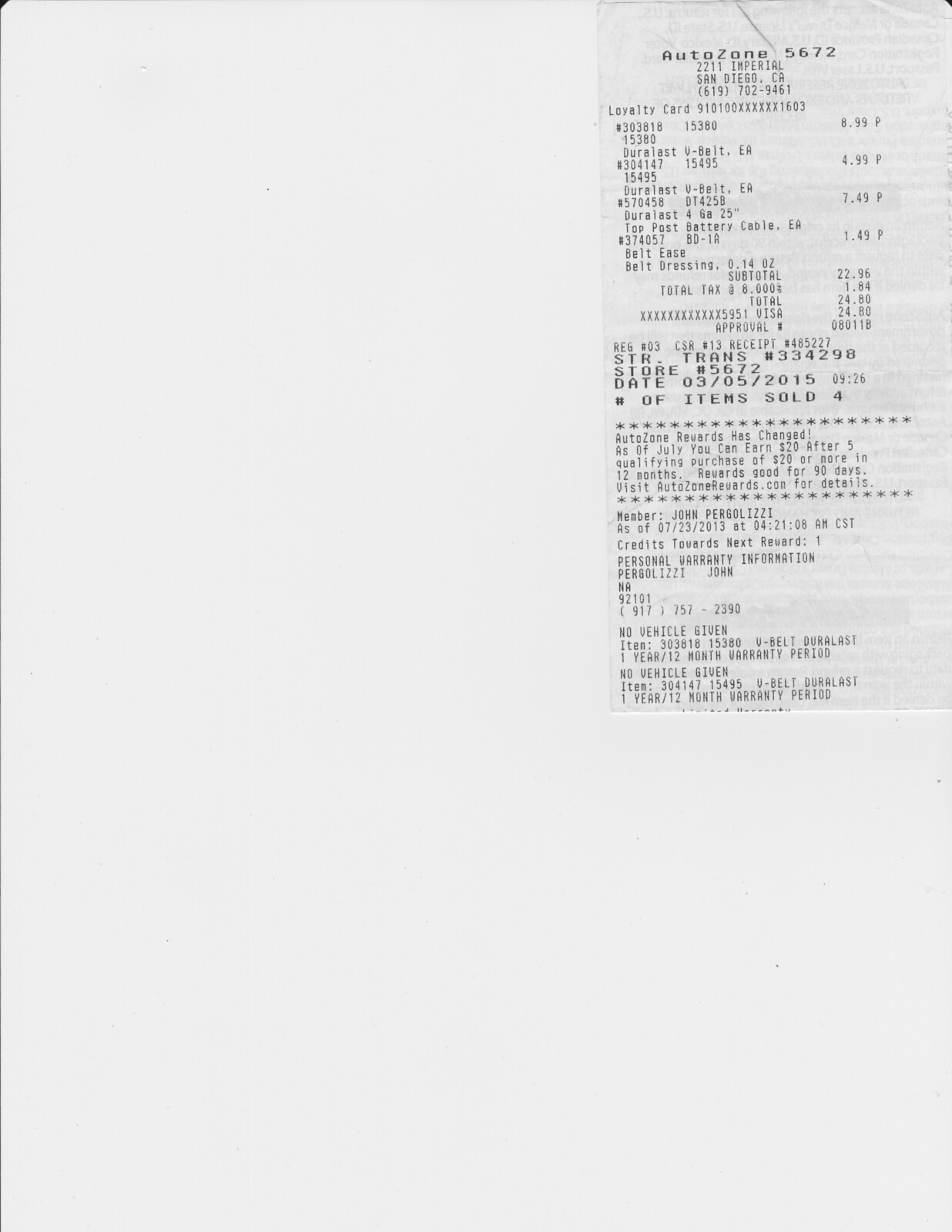This is a scanned black and white photocopy of an AutoZone receipt. The receipt is from AutoZone store number 5672, located at 2211 Imperial, San Diego, California, 619-702-9461. Purchased items include two Duralast V-Belts, one Top Post Battery Cable, and one Belt Dressing, with a subtotal of $22.96. After tax, the total comes to $24.80, paid via Visa card. The receipt details a transaction made by a customer named John Persolizzi on March 5, 2015. The receipt includes typical store information, loyalty card number, and is primarily used for reference or business purposes such as tax documentation.